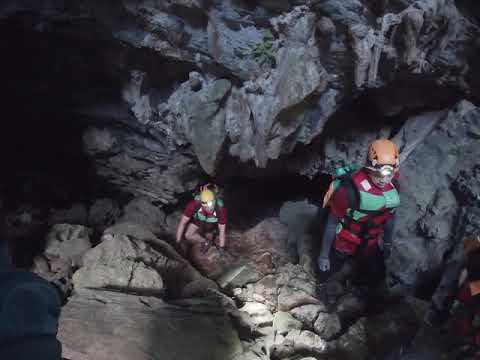This detailed landscape-oriented color photograph captures an interior view of a dark cave illuminated solely by the headlamps of two spelunkers. In the foreground, a person of likely brown skin with an orange hard hat featuring a central light, a red short-sleeved shirt over a long-sleeved black shirt, and a backpack with green and black straps, attentively walks on a rocky, uneven path. Their gaze is fixed downward to avoid tripping over the numerous loose rocks strewn across the ground. Just behind, a second explorer, of Caucasian descent, navigates the rough terrain. He wears a yellow hard hat equipped with a headlamp and a short-sleeved red shirt paired with shorts. He is seen using his hands and one knee to climb up natural stone steps, carefully maneuvering through the tight space with jagged overhead formations that restrict movement. The rocks, in shades of dark and light gray, form a dramatic natural landscape that is mesmerizingly lit by the explorers' lamps, highlighting the arduous ascent within this vivid scene of realistic photographic representationalism.